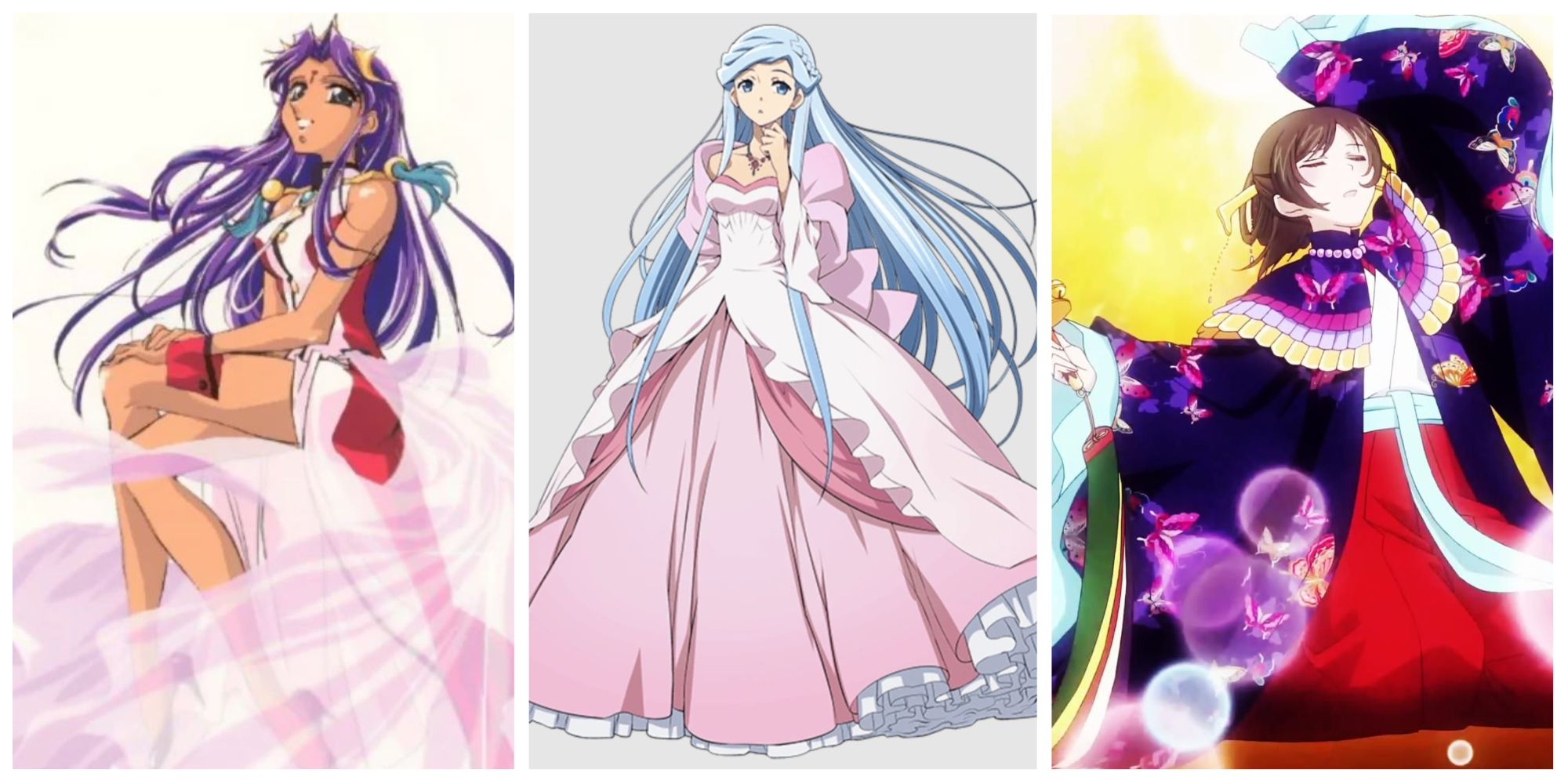The image features three distinct anime characters, each occupying a triangular section of the composition. On the left, there is a woman with long purple hair and large, expressive eyes, characteristic of anime style. She dons a red and white short outfit with a veil, and the background behind her is light yellow. In the center, a girl with light blue, dual-shaded hair stands out in her floor-length pink gown adorned with white frills and petticoat, set against a light gray background. To the right, another girl is shown, this time with short brown hair styled in a bun. She is dressed in a white and red kimono with a purple outer robe, displaying varying shades of purple from dark to lavender, and her eyes are closed, giving her a thoughtful demeanor, all set against a yellow background.